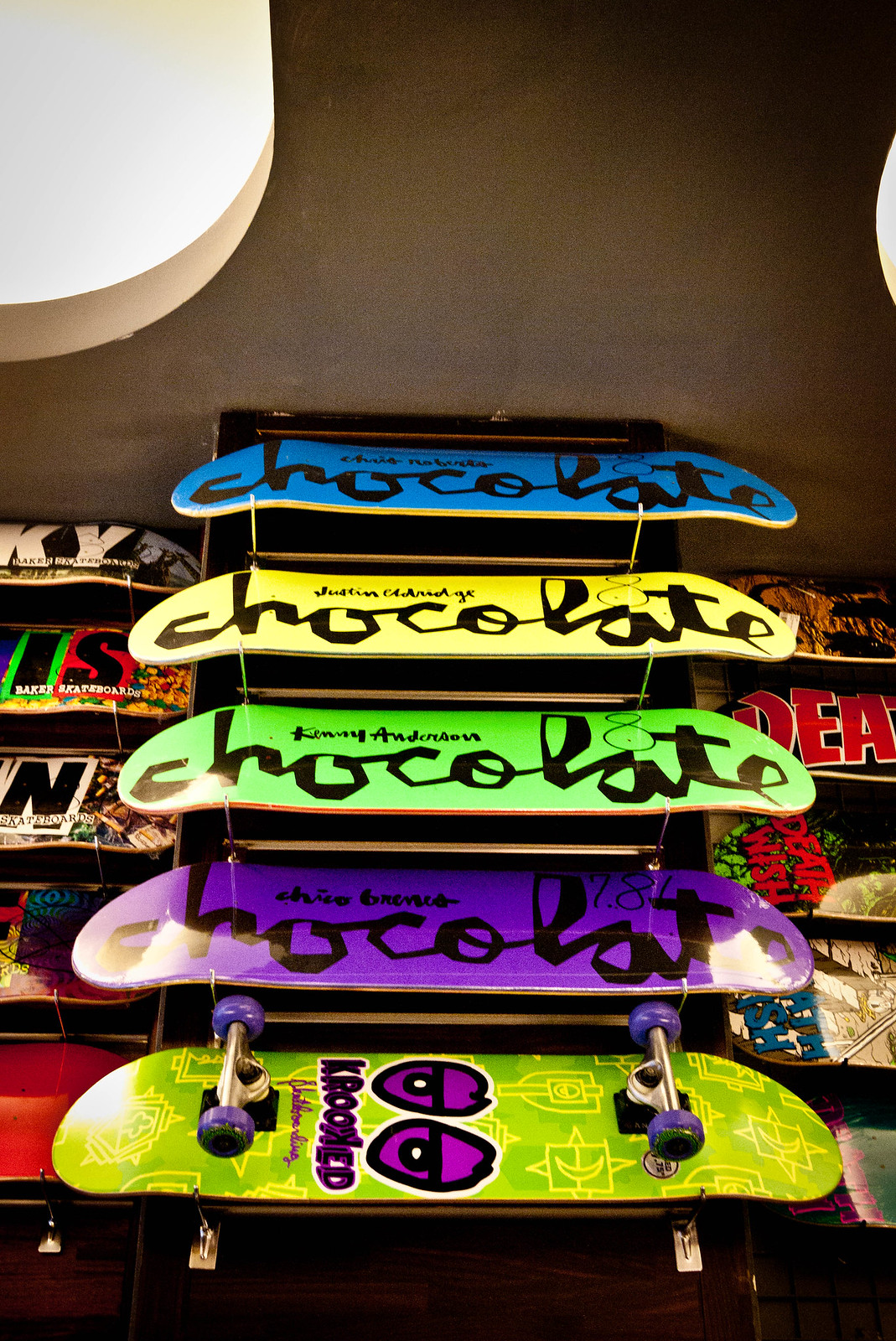This photograph, likely taken inside a shop, provides a slightly overhead view of a display of skateboards against a dark brown wall featuring cutouts that reveal light blue or white in the background. The display showcases ten skateboards arranged in racks. On the left, half of five skateboards are partially visible, while on the right, the ends of another five skateboards come into view, some featuring graffiti-style text with phrases like "Death Wish" and "Death."

Central to the display, a taller black rack holds five skateboards in a staggered arrangement. The top skateboard is blue with the word "chocolate" in black cursive, followed by a yellow skateboard, then a green one, and a purple one—each also bearing the word "chocolate." At the bottom of the rack is a lime-green skateboard adorned with yellow cartoon designs and a pair of purple eyes looking left, along with purple lettering spelling "crooked" with a K. This skateboard is unique in the display as it is the only one featuring wheels, which are purple.